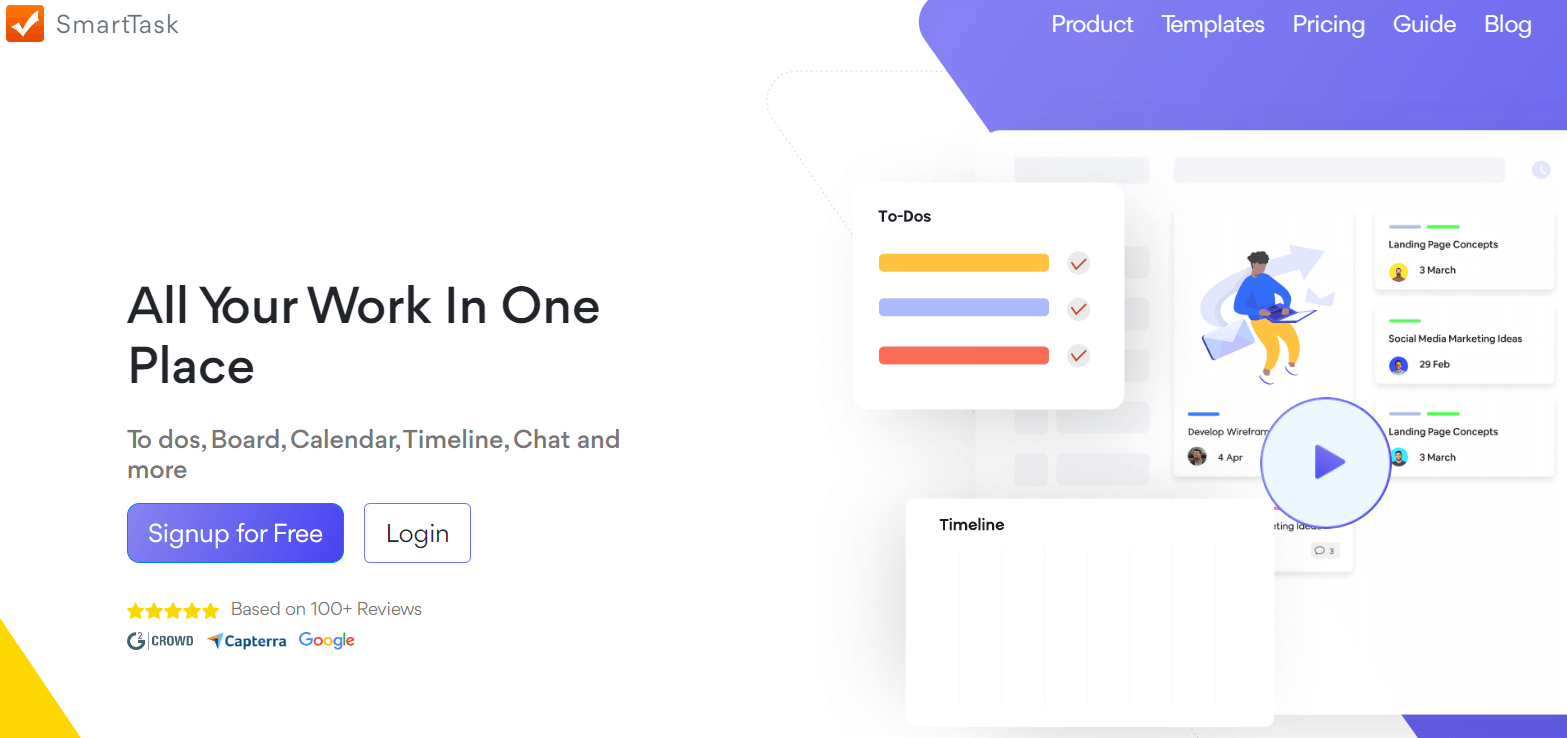**Smart Task Website Homepage Overview**

The website homepage of Smart Task, a productivity and project management company, features a vibrant and well-organized layout. Prominent on the left side is the company logo represented by an orange box with a white check mark inside.

On the right, there is a purple navigation bar with white text, showcasing sections labeled: "Product," "Templates," "Pricing," "Guide," and "Blog." Below this navigation bar is a bold headline in large black letters stating, "All your work in one place." Beneath this headline, a list of features is displayed, including "To-dos," "Board," "Calendar," "Timeline," "Chat," and more.

At the center of the page, there is a prominent call-to-action with a purple oval-shaped button saying "Sign up for free." Next to it, a white box invites users to "Log in." Directly below these buttons are five gold stars indicating a high rating, supported by "100+ reviews."

Further down, the page mentions a partnership with Google and another sponsoring company, although their details are not specified. In the top left corner of the page, there is a small gold triangle accent.

On the right side of the page, a detailed section is presented showing active to-dos, featuring a gold bar, a blue bar, and a red bar, each with check marks. An engaging image illustrates a man wearing a blue shirt and gold pants, working on a laptop. He appears to be moving an envelope, symbolizing task management.

Additionally, there is a purple-outlined white circle with a purple arrow, which, when clicked, plays an explanatory video. This video provides insights into the workings of the platform. The page is segmented into different categories, with a significant focus on the "Timeline" section, offering a comprehensive view of project timelines.